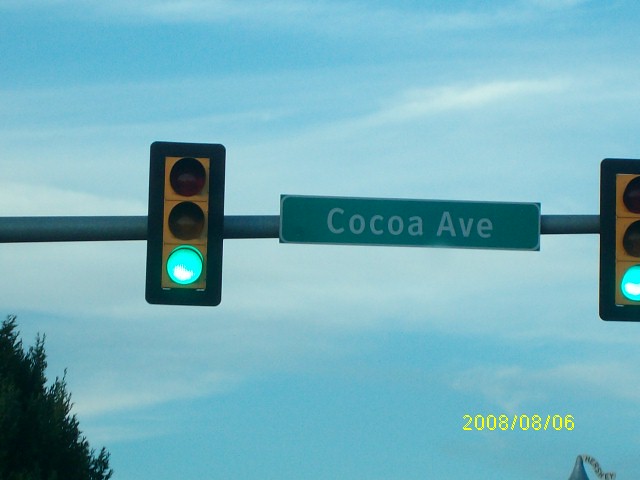In this detailed outdoor daytime photograph, a horizontal dark green or black metal post stretches across the scene, supporting two traffic lights - one on the left and one on the right, both illuminated with green lights. Centered between these traffic lights is a green street sign with white lettering that reads "Cocoa Avenue." The background features a clear blue sky with wispy white clouds, adding a serene atmosphere to the image. On the far left, the silhouette of an evergreen tree is faintly visible. In the bottom right corner of the picture, stamped in yellow, is the date "2008-08-06." Additionally, a Hershey's Kiss, colored in silver with a white tag reading "Reese's," can be seen partially in the bottom right corner, making a subtle nod to the famous chocolate brand.